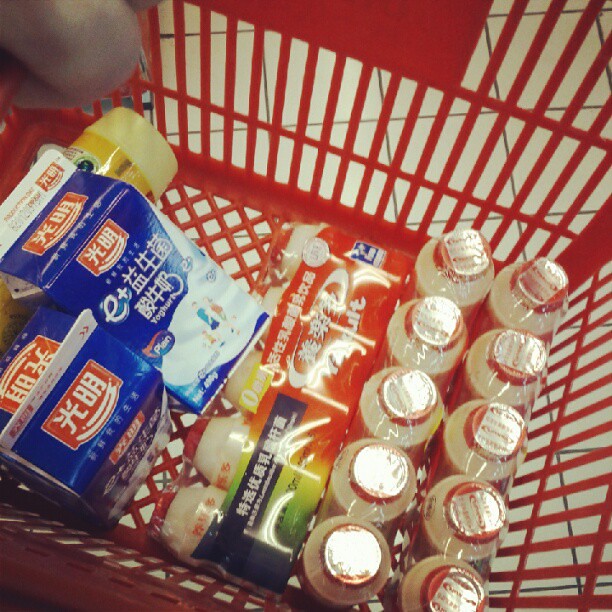In this image, you see a red plastic shopping basket featuring a distinct design: the bottom has a pattern of small diagonal squares, while the sides have longer rectangular holes. The basket contains various grocery items, predominantly Asian food products. Inside, there are three packages of Yakult yogurt drinks; two are standing upright next to each other, and one is lying on its side. These drinks have off-white bottles with red caps and silver foil seals, packaged in red, green, and white wrapping that includes Chinese characters.

Additionally, the basket holds two small cartons of milk, which are blue and red with designs that include white spilled milk imagery and Chinese writing. There is also a cylindrical yellow item, potentially shampoo or a different type of drink, with a matching yellow top. The photo is taken from above, revealing beige floor tiles below the basket. A small portion of a person's bent finger is visible at the top left corner, indicating they are holding the basket.